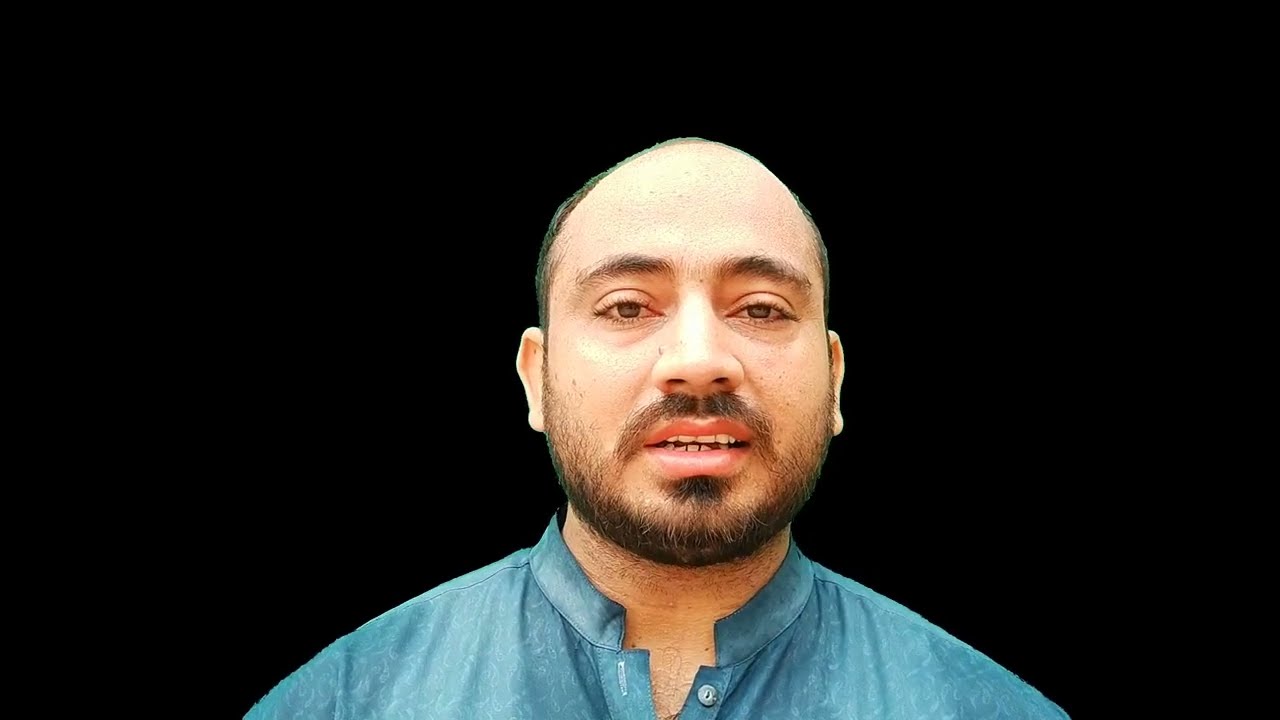In this image, a man sits against a completely black background, his presence stark and isolated. He is wearing an aqua blue button-down shirt with a subtle white swirly pattern and a dark blue button, though the image cuts off at his shoulders, leaving the full design of the shirt unseen. The shirt has a unique pop-up circular collar instead of a traditional one. The man has a bald head, and his receding hairline features some black hair growing onto his neck. His face is marked by bushy brown eyebrows and a thickening brown beard and mustache, with a distinctive patch of facial hair under his bottom lip. His mouth is slightly open, as if caught mid-speech, suggesting the image is a still from a video, possibly an instructional or testimonial one. His eyes, brown with a slightly pink haze, convey a sense of sadness. There are no additional elements in the image—no text, tattoos, or earring—just the man centered in the frame, gazing directly at the camera.